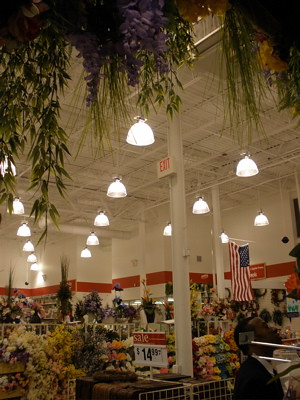The image depicts the interior of a bustling retail store, teeming with greenery and vibrant colors. Suspended from the ceiling are an array of lush, hanging plants, their verdant foliage cascading downward, creating a natural canopy. The ceiling itself is constructed from sturdy metal beams, adding an industrial flair to the space. Attached to the beams are numerous bright white lantern-style lights, illuminating the area with a soft, yet brilliant glow. 

In the background, a large American flag is prominently displayed against the far wall, adding a patriotic touch. The walls are a pristine white, interrupted by a striking bright red stripe that runs horizontally at mid-height, injecting a burst of bold color.

In the foreground, an assortment of flowers is artfully arranged for sale, their blossoms adding a riot of color and life to the scene. Perched on a white pole, a sale sign reads "Sale $14.99," indicating a special promotion on the various kinds of flowers available. The overall ambiance of the store is a harmonious blend of industrial elements and vibrant natural beauty, inviting and visually dynamic.